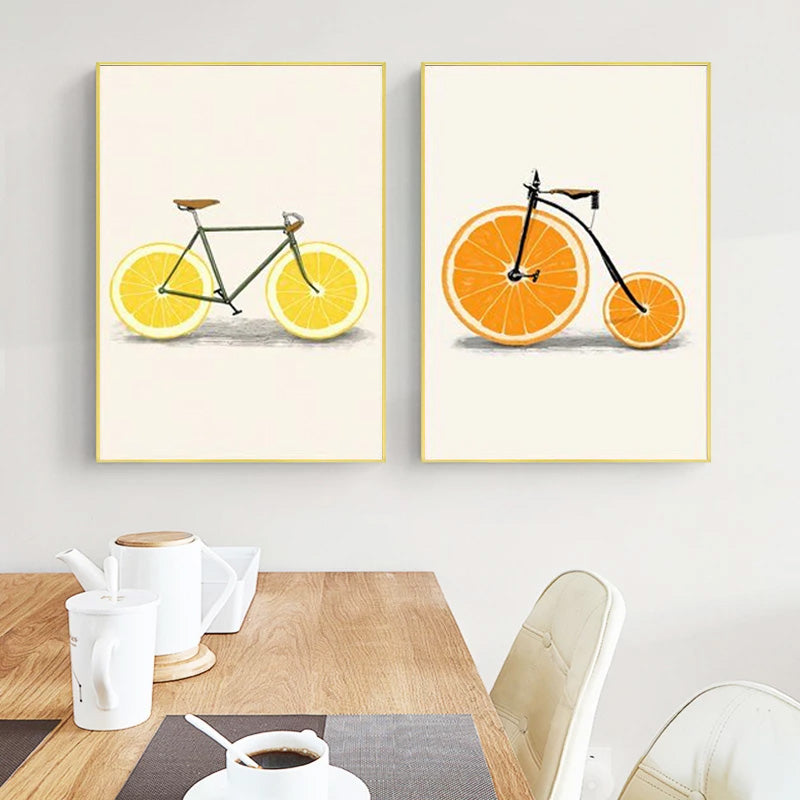A detailed photograph captures the interior of a room, drawing attention to a white wall adorned with two distinctive rectangular paintings. Each painting features a whimsical bicycle, with one on the left having wheels fashioned from yellow lemon slices and the one on the right showcasing a vintage bicycle with wheels made from vibrant orange slices. Positioned in front of this artful backdrop is a wooden table, partly visible and brown in color. The table is set with an array of items including a white coffee cup filled with coffee, accompanied by a white spoon and saucer resting on a two-toned gray mat. Additional items include a teacup or another coffee cup, a likely sugar-filled cup, and a white tray. Flanking the table are several white chairs, strategically placed in the bottom left and right corners of the image, completing the serene and thoughtfully arranged indoor scene.